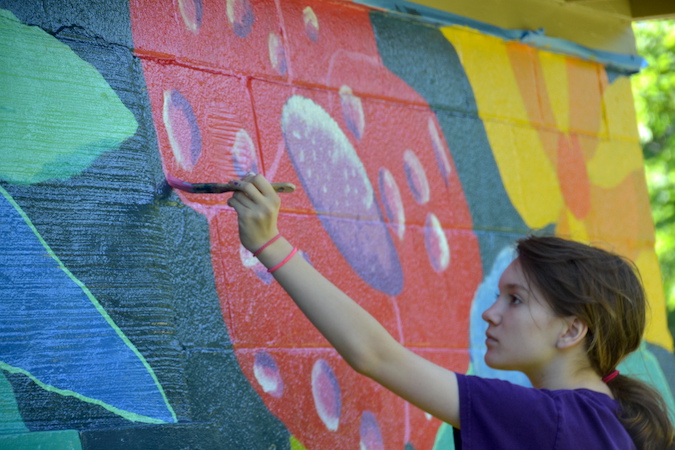In this close-up, outdoor photo, a young girl is captured in the act of painting a vibrant mural on a cinder block wall. The wall serves as a canvas with a fully painted green background adorned with large, colorful flowers. The girl, who appears to be about 15 years old, is intently focused on her work as she outlines a central red flower with a pink paint. She is right-hand dominant, her left hand is raised and steadying herself against the wall. Her light skin contrasts with her blue short-sleeved t-shirt, and she accessorizes with two distinct pink bracelets on her wrist. Her long brown hair is styled in a loose ponytail, keeping it out of the way as she meticulously applies the pink color using a thick paintbrush. The mural also features a large yellow flower with an orange center and parts of blue and green flowers to the left. In the top right corner of the image, the tops of trees can be seen beyond the building, adding to the outdoor daytime setting.